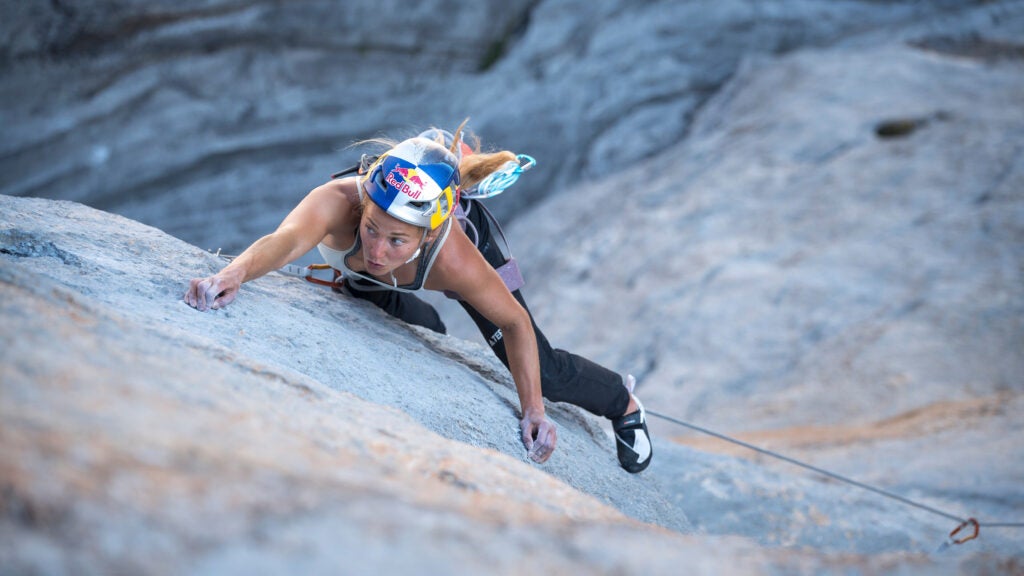In this horizontally aligned, rectangular image, a woman with slender, tanned, and muscular arms is rock climbing up a steep, almost vertical rock face. She is at the center of the photo, and we are looking down at her from above. Her chalky hands are gripping the rock, which is largely gray with hints of brown, especially noticeable in the lower corner. The rock formation features large ledges, particularly on the right side, with a blurry section on the upper left. The climber is secured with a rope that extends downward towards the lower right, with a visible clip attached to it.

Dressed in a white and gray tank top and black pants, she also wears a blue and white helmet with the Red Bull logo in red. Her blonde hair is pulled back, tucked under the helmet. The photo captures her in the act of climbing, showcasing her harness and climbing shoes. The steepness and height of the climb make the scene appear both dramatic and daunting.